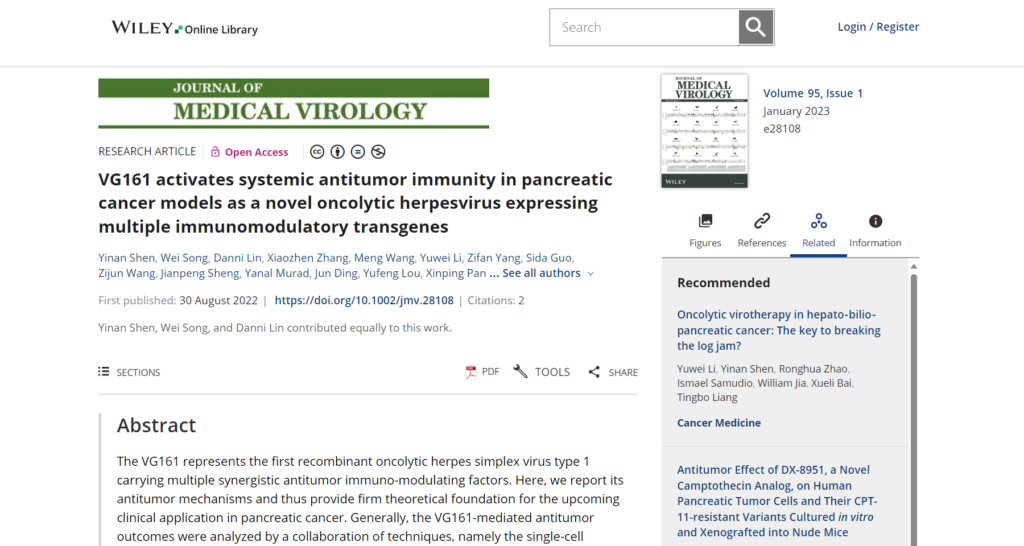The image depicts the Wiley Online Library homepage. At the top, a dominant white bar extends across the width of the page. On the left, the Wiley Online Library name is displayed alongside a green and black logo. To the right, there's a search box with a gray search button, followed by options to log in or register. Just below this, a thin gray line separates the top section from the content below.

On the left side of the main content area, a green section of text reads "Journal of Medical Virology." Below this heading, an article is listed, accompanied by buttons for tools, PDF access, and sharing options. Additionally, there's a 'Sections' button next to the article title.

This article is identified as a "Research Article" and is marked "Open Access" in pink. An abstract of the article is provided underneath. On the right side of the page, the volume and issue number, "Volume 95 Issue 1," are displayed at the top. Below this, there are buttons for "Figures," "References," "Related," and "Information." At the bottom right of the page, a "Recommended" section is included, likely suggesting related articles or content.